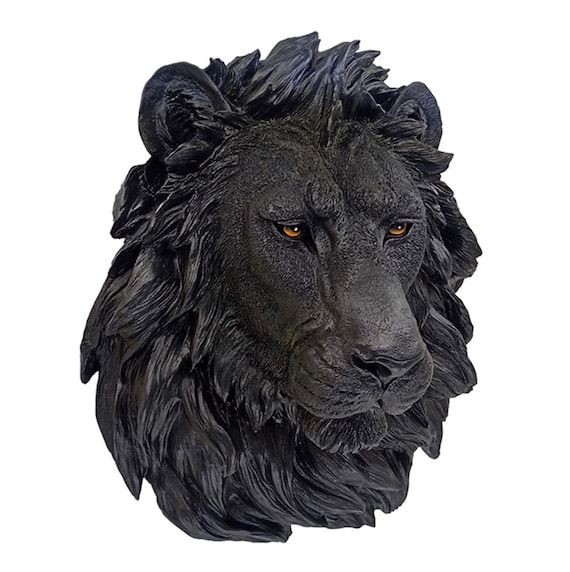This image showcases a highly detailed sculpture of a male lion's head, set against a plain white background. The sculpture is crafted from a black material with grey highlights that accentuate the intricate details. Each strand of the lion's mane is meticulously defined, making the texture of the fur highly realistic. The lion's face bears a frowning expression, with its mouth closed and eyes looking slightly to the right. The eyes are a striking yellow-brown (orange) with black pupils and a reflective glint of light, adding to the sculpture's expressive quality. Despite the dark tones of the sculpture, the high level of detail in the snout, mane, and facial features is clearly visible, highlighting the craftsmanship involved.